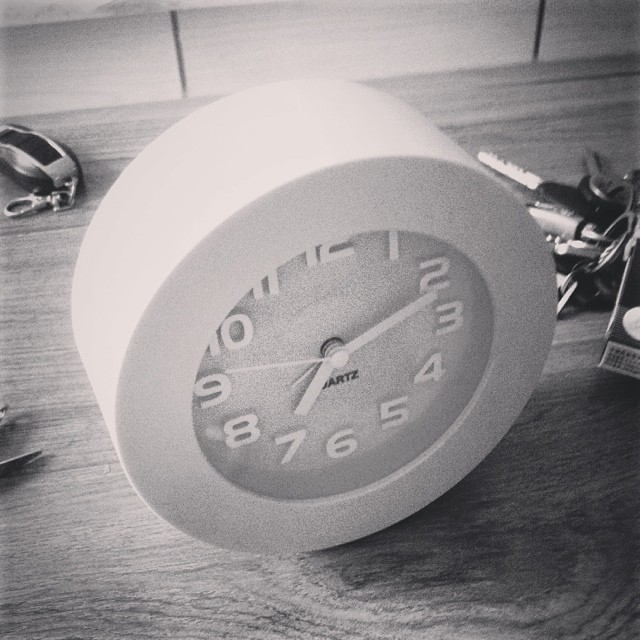This black and white photograph captures a close-up of a classic round white quartz alarm clock sitting on a wooden bedside table, presumably made of oak with visible grain. The clock displays a time of approximately 7:11:47, with black letters and the word "quartz" underneath the hands. Next to the clock is a set of keys, and behind it lies a black and silver keychain. Additionally, a pair of tweezers or perhaps scissors is partially visible to the left. The scene is framed by a tiled wall in the background, adding texture to the monochromatic composition.